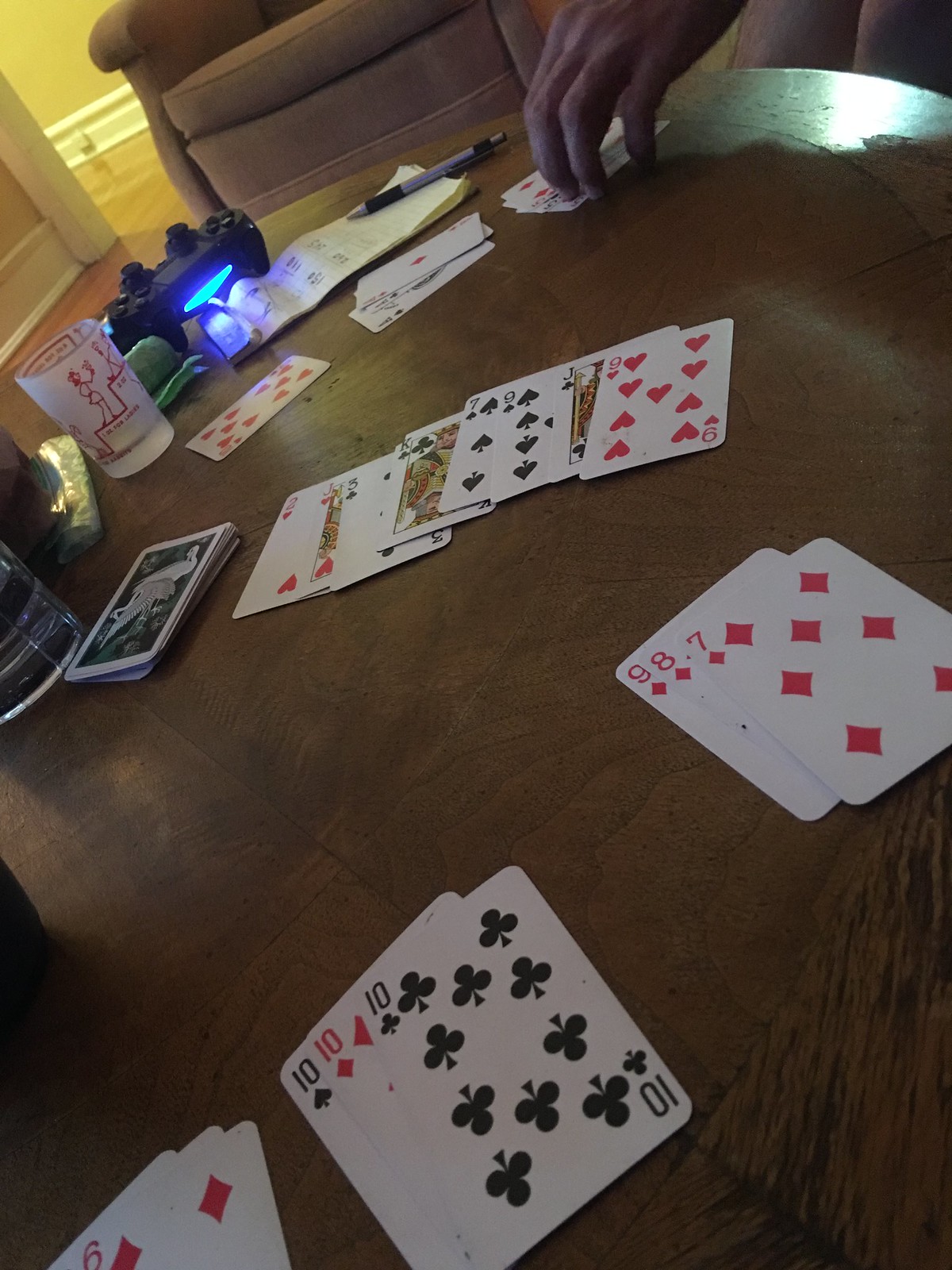The photo primarily features a dark wood table covered with an array of playing cards, suggesting a game of poker in progress. In the far upper left corner, a glimpse of a white wood floor is visible, along with a hint of a yellow wall that appears to turn around a corner. Next to this corner stands a dark-colored couch. On the upper reaches of the couch arm, there is a game controller, possibly from a PS5 or Xbox, alongside a notepad with a pen resting on it.

In the lower part of the image, immediately below the couch arm, a hand can be seen holding or resting on a set of cards on the table. Across from this hand, a transparent shot glass is noticeable. Scattered around the table are several other cards, including a specific stack with eight cards laid out.

Closest to the camera are three notable hands of cards: one features the nine, eight, and seven of diamonds, and another includes three tens (spades, diamonds, and clubs). Additionally, towards the left corner of the image, three more cards are present, with the six of diamonds being identifiable.

In the middle left of the frame, a partially visible glass dangles off the edge of the table, but no further details about the glass can be discerned. Overall, the scene is vibrant with activity, capturing the essence of a lively card game.